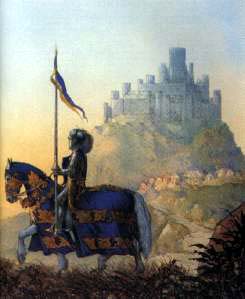This detailed painting depicts a medieval scene with a knight in shining armor riding a horse, set against the backdrop of a grand castle atop a verdant mountain. The castle, painted in muted gray and blue hues, features numerous cylindrical towers, including a prominent central tower that stands tall. The mountain, adorned with lush greenery and a winding, sand-colored path, enhances the majestic atmosphere. 

In the foreground, the knight, clad in full armor, holds a flagpole with a blue and yellow flag. The knight's steed, also elaborately dressed, wears a long, royal blue blanket with golden accents. The horse, lifting its left front leg, appears poised as it moves through the grass. The sky behind the castle transitions from a deep blue at the top to a warm orange closer to the horizon, adding a dramatic effect to the scene. The overall image, rendered in a somewhat blurry, low-resolution quality, captures the essence of medieval chivalry and grandeur.